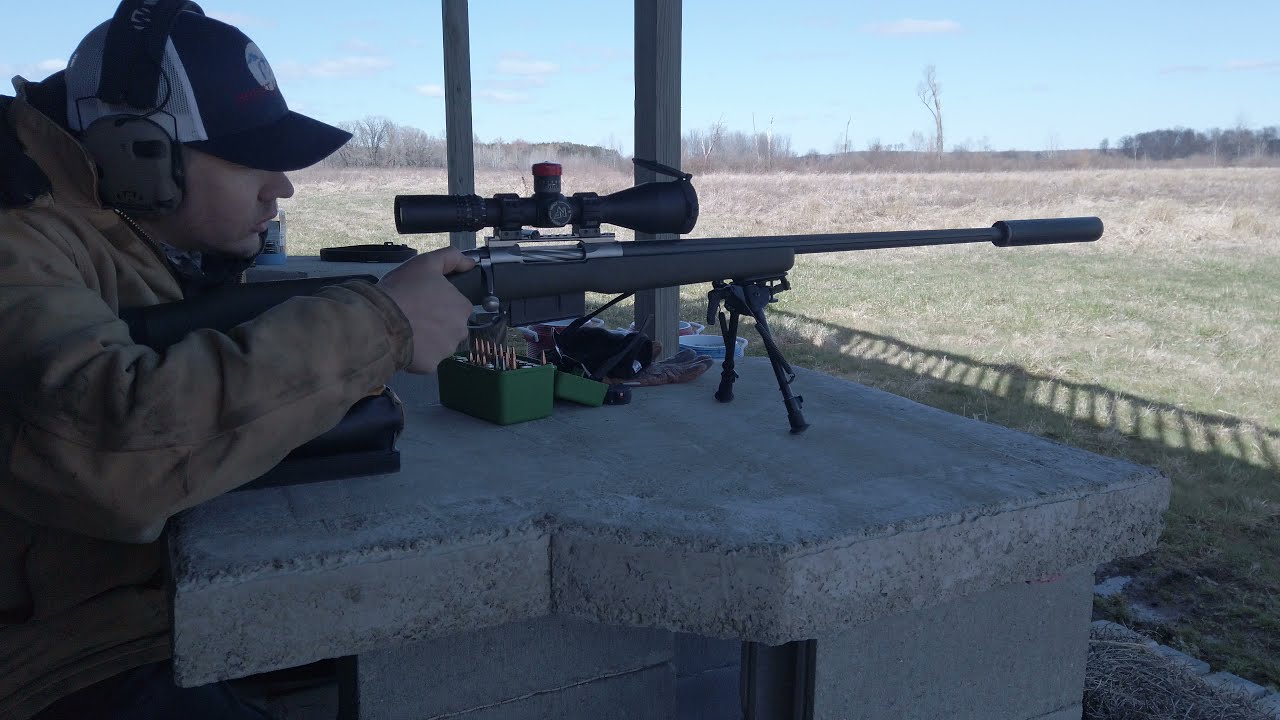The image depicts a Caucasian man intently positioned at a shooting range, preparing to fire a rifle mounted on a stand atop a concrete table. He is sitting comfortably behind the table, which is laden with shooting accessories including a green box of ammunition, cleaning supplies, and various other gear. The man, wearing ear protection and a blue and white ball cap that partially obscures his eyes, is dressed in a well-used, beige-toned jacket that looks grimy, possibly from black powder. His right hand is poised on the rifle, which features a scope and potentially a suppressor at the end. His arm rests on an armrest attached to the table, providing stability as he peers through the scope. The expansive field in front of him is devoid of other people or structures, extending to the horizon where scattered thin trees and puffy white clouds punctuate the blue sky. Shadows suggest there might be a second story or overhang above him.